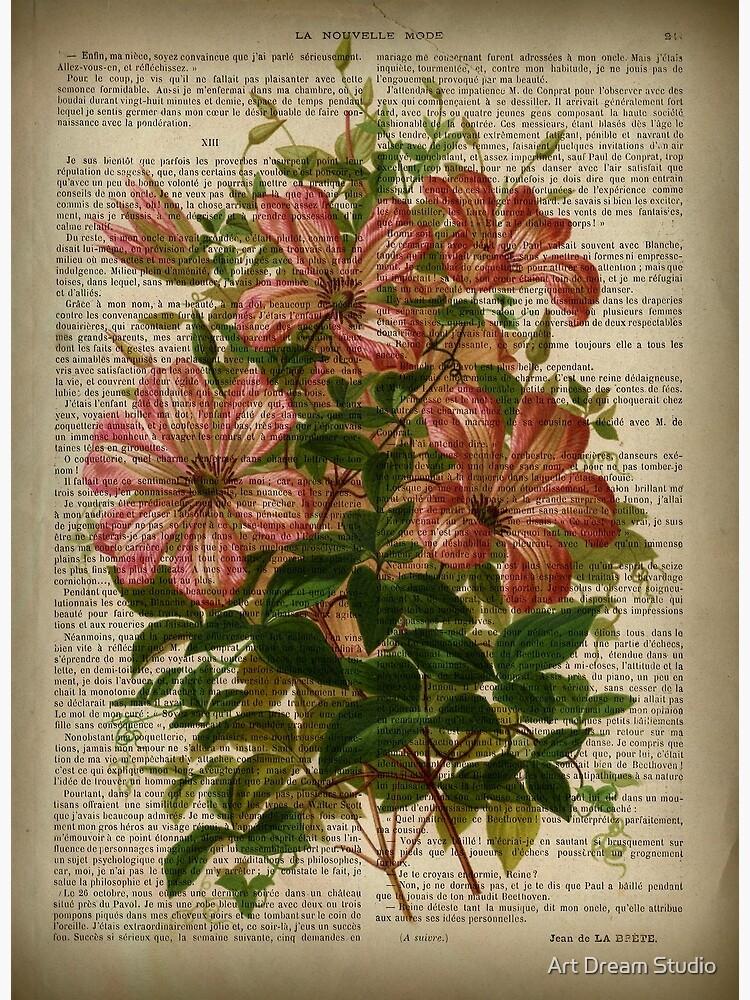The image features a vintage-looking page from a book, titled at the top "La Nouvelle Mode," indicating its French origins. The aged, brown paper is covered in fine, small lettering that appears to be text from a novel or magazine. Overlaying the text is a detailed, textured drawing of daylilies. The daylilies exhibit a gradient of pink on the edges of their petals fading to a lighter pink or white at the center. Brown pistils and green leaves are visible among the flowers, adding to the ornate and delicate appearance. There are seven daylilies in total, depicted in various stages of bloom. The stems and foliage spread organically across the page, merging with the text to create a harmonious composition. The bottom right corner of the page bears the phrase "Art Dream Studio" in small, white letters, adding a final artistic touch to the vintage illustration.